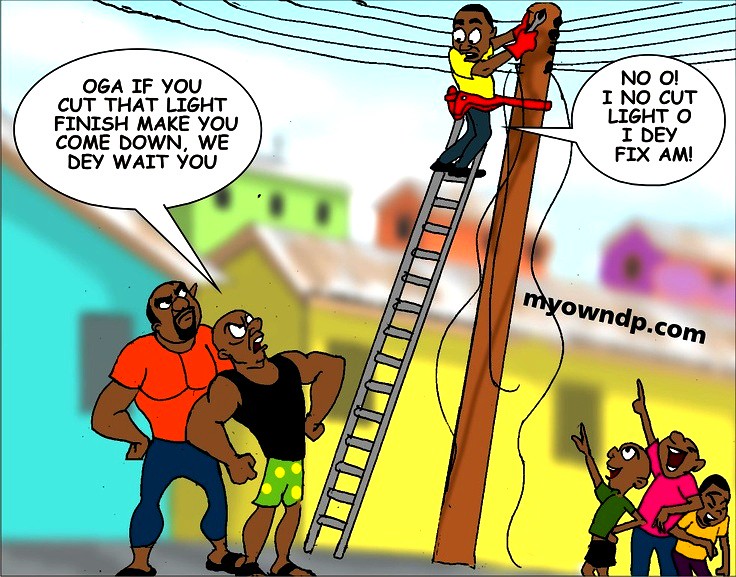This image is a colorful, cartoon-style comic strip panel set in an urban landscape. The scene features a man centered at the top of the illustration, climbing a ladder and working on electrical equipment attached to a telephone pole. He appears nervous as he looks down. Below him, two muscular African men on the left, looking perturbed, are saying, "OGA, if you cut that light, finish make you come down, we dey wait you." The man on the ladder, in response, is saying, "No, oh, I no cut light, oh, I dey fix am."

To the bottom right, a crowd of younger people are pointing and laughing at the man on the ladder. The entire scene is vibrant and colorful with an assortment of colors such as blue, tan, white, black, orange, green, yellow, brown, purple, and pink, seen in both the background buildings and the clothing of the characters. The background, though blurred, reveals a skyline of colorful buildings set against a sky, adding depth to the illustration. The piece includes a URL, "MyOwnDP.com," printed on an angle to the right. This lively cartoon captures a humorous yet tense moment, set against a vivid and bustling urban backdrop.